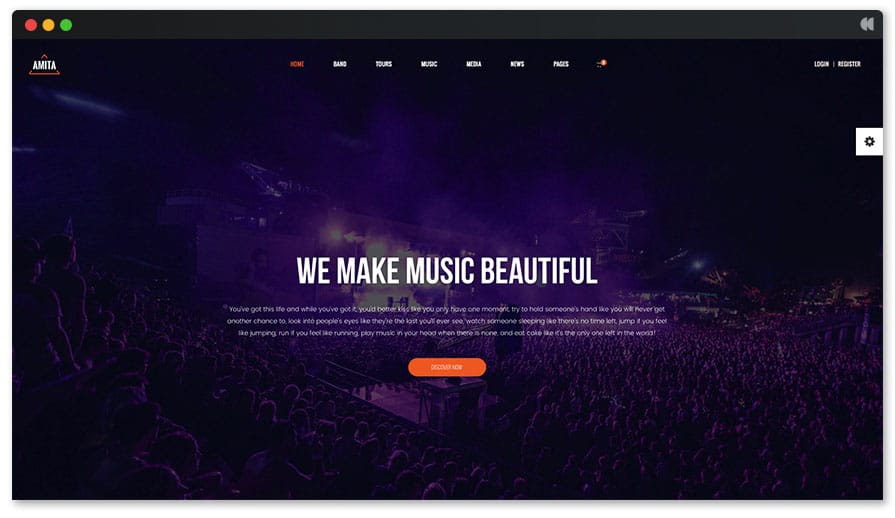This screenshot from a music-themed website showcases a sleek and visually engaging layout. At the top, a black navigation bar features three colored dots—red, yellow, and green—on the left side, resembling a typical window control interface. Adjacent to these dots is the website’s logo, which features "AMITA" in white text, encased in an orange triangle.

The navigation bar includes several menu options: Home, Band, Tours, and others that are indistinguishable, accompanied by the Login and Register buttons, facilitating user interaction. Below this bar, the bold, uppercase text declares, "WE MAKE MUSIC BEAUTIFUL," likely the site’s tagline or mission statement. Beneath this powerful proclamation, a brief paragraph in white text offers additional information, although details remain unclear.

Centrally positioned, a prominent orange button with white text invites further engagement, though the specific call-to-action is not legible. Dominating the visual space is an image capturing the vibrant atmosphere of a live music event. While the performers are not visible, the crowd and stage are clearly depicted, suggesting either an indoor venue or an outdoor night event.

Overall, the screenshot effectively conveys the site's focus on music and live events, drawing users into its dynamic world.